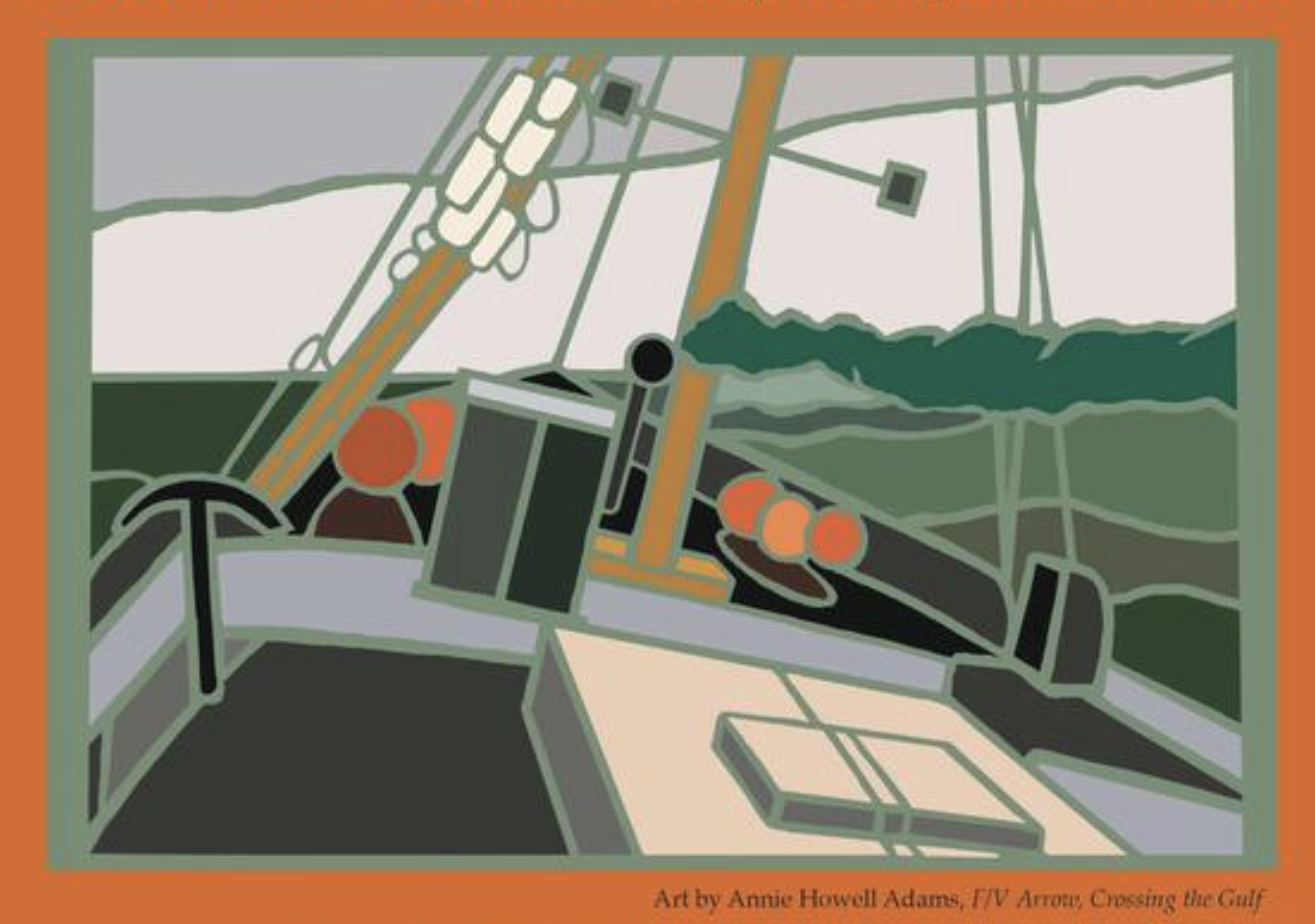This detailed painting by Annie Howell Adams, titled "FV Arrow Crossing the Gulf," features a modernistic portrayal of the interior of a sailboat. The square composition is rendered in shades of green, gray, orange, white, black, and hints of peach or pink. The scene illustrates the top deck of a sailboat slightly tilted to the right, perhaps 20 degrees, showcasing the lower part of the mast and the open deck. On the deck, details include a white-painted hatch, a miner's pick, and a control box with a black lever. The surrounding seas appear dark and somewhat rough, contrasting with the vibrant deck details. The vessel seems to be in motion, with simple outlined figures suggesting crew members. The artwork evokes a sense of rugged maritime adventure through its modern art style and dynamic composition.